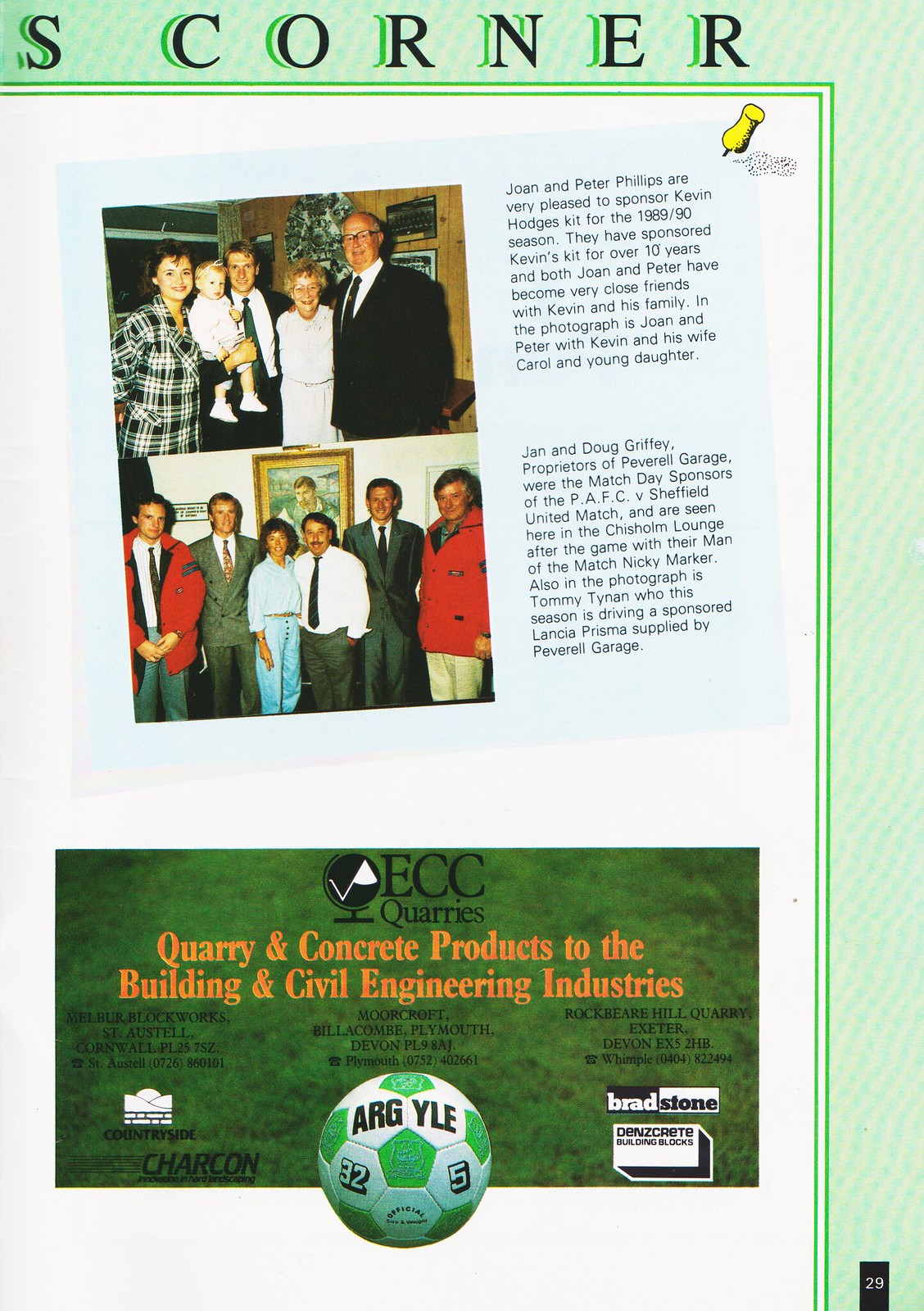The image is a scan of a page from a soccer magazine featuring a light green background with green and white wavy stylization resembling a pinned note. At the top of the page, the title "S. Corner" is prominently displayed in large font. The page includes two family portraits along with descriptive paragraphs explaining their sponsorship activities.

The top portrait shows Joan and Peter Phillips with Kevin Hodges, his wife Carol, and their young daughter. The accompanying text reveals that Joan and Peter Phillips have been sponsoring Kevin Hodges' kit for the 1989-90 season and have maintained a friendship with his family for over a decade.

The second portrait features Jan and Doug Griffey, proprietors of Peverell Garage, who were match day sponsors for a PAFC versus Sheffield United game. They are pictured in the Cristone Lounge with their man of the match, Nicky Marker, and Tommy Tynan. The text highlights that Tommy Tynan is driving a sponsored Lancia Prisma supplied by Peverell Garage.

Below these family portraits, there is an advertisement for Corian Concrete Products, emphasizing its services to the building and civil engineering industries. This section of the magazine is marked as page 29, indicated by a small number in the bottom right corner.